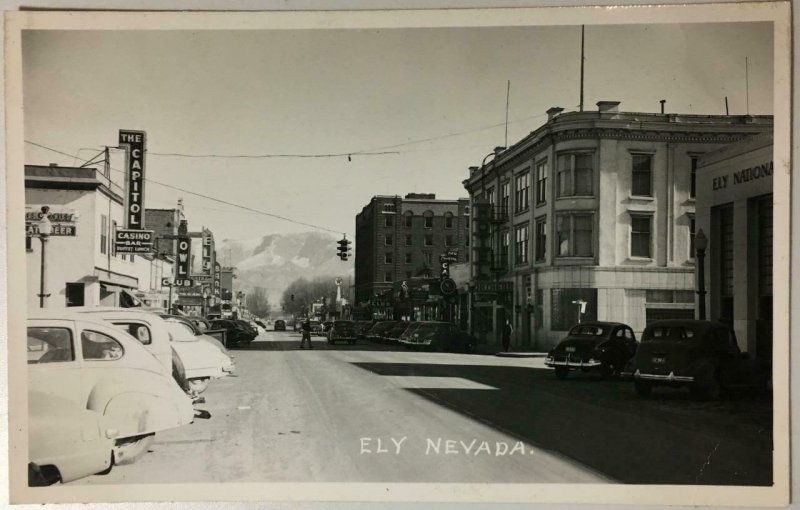This is an old, black-and-white photograph of Ely, Nevada, likely taken in the 1940s or 1950s, suggested by the vintage style of the parked cars. The faded hues of yellow, black, and gray give the image an antiquated look. The picture captures a street view with buildings flanking both sides: the left side hosts a series of establishments, including the National Capital Casino Bar and the Owl Club, adorned with neon signs. The right side features primarily businesses and a prominent sign for ELY National Bank on a government-like building. The street is populated with numerous old-time cars parked along the sidewalks and includes several streetlights at intersections, with at least three visible down the road. In the distance, the street leads the eye toward a backdrop of majestic mountains. A small white inscription at the bottom of the photo reads "ELY, Nevada." The scene portrays the blend of commercial vibrancy and the classic charm of this Nevada town.